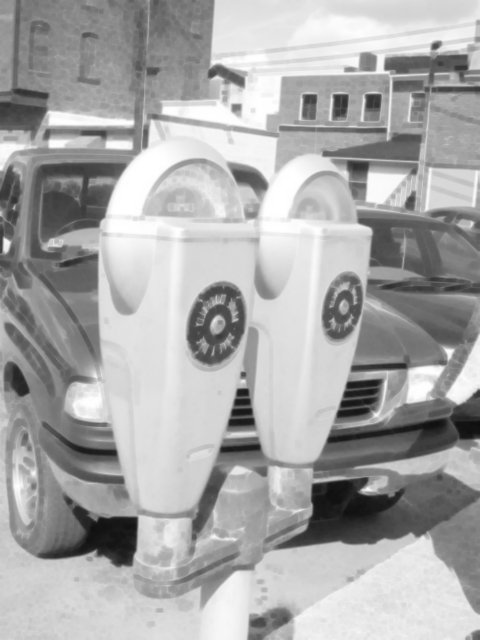This black and white photograph, likely taken a long time ago, captures an urban street scene featuring two vintage parking meters mounted on a single pole. The meters, which extend from either side of a white pole and are connected by a gray metal piece, boast a black circle in the middle and a clear glass panel bordered by white at the top. In the foreground, a dark-colored car with black tires and white headlights is parked facing the perspective of the photo, with another similarly colored car adjacent to it. The scene is set against a backdrop of various buildings: a tall stone building to the left, shorter brick structures with dark windows to the right, and one building with a pipe running up the side. The urban landscape is further detailed with visible power lines and a dark roof. The sky appears gray with some white clouds, adding to the historic feel of the photograph. The sidewalk in front of the parking meters sets the stage for this nostalgic glimpse into a bygone urban environment.